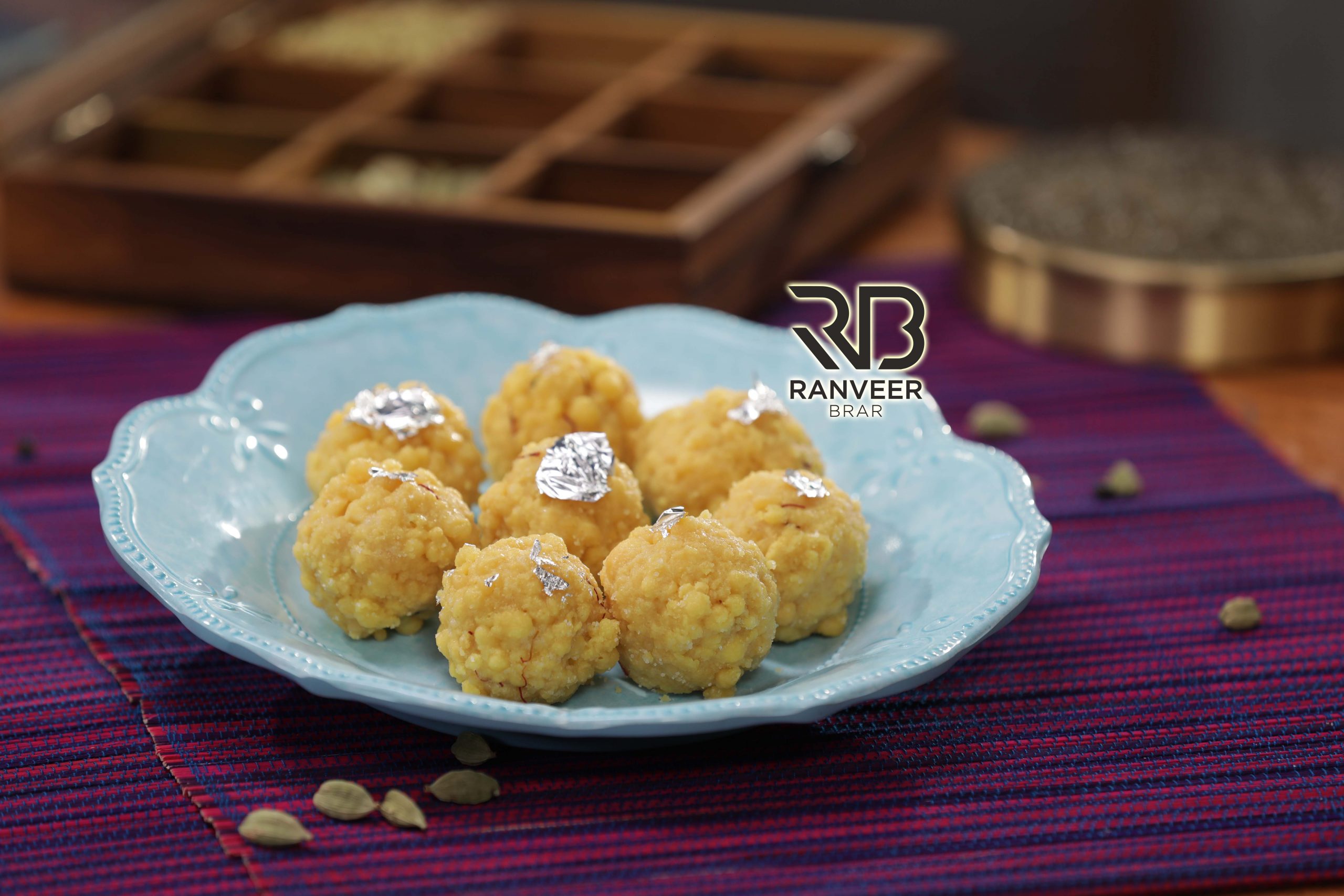On a rustic wooden table adorned with a red and purple checkered tablecloth, there sits a light blue glass plate with a gently curved rim. The focal point of the image is the dish on this plate, which features eight round, yellowish balls reminiscent of cauliflower in texture. Each of these meticulously crafted balls has a small piece of tinfoil delicately placed on top. Surrounding the plate on the tablecloth are scattered peeled sunflower seeds, adding a touch of natural texture to the scene. In the blurry background, a wooden tray with nine separate compartments is visible, holding a gold circular tin, possibly filled with more of the sunflower seeds. The image is subtly watermarked with the logo "RB" in a sophisticated font, with the name "Ranveer Brar" elegantly inscribed beneath it.